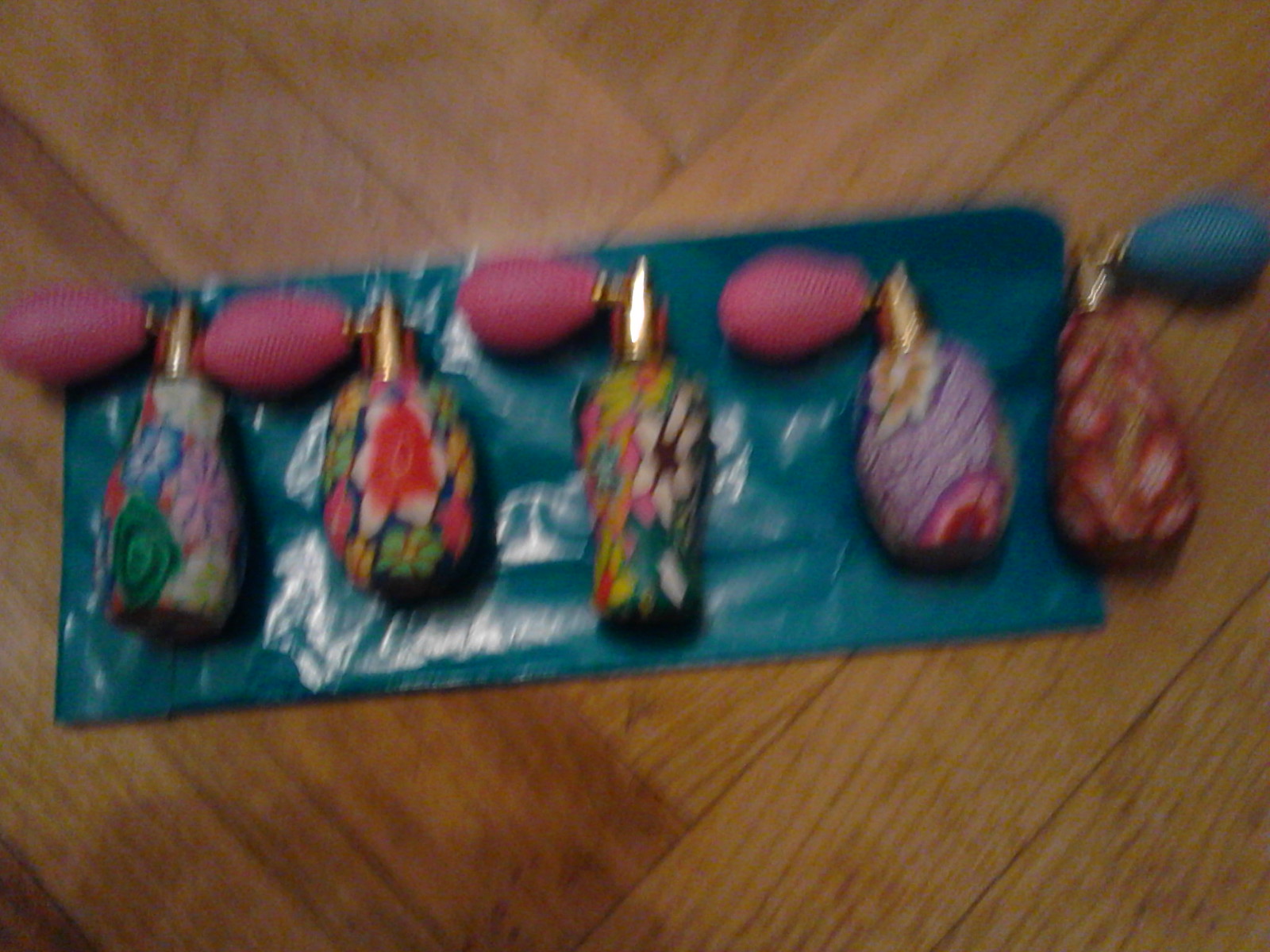This blurry image depicts five perfume bottles arranged in a line from left to right, positioned on a light brown, wooden floor that shifts from horizontal planks on the right to vertical on the left. The bottles rest atop a bluish, teal plastic bag. Each perfume bottle is adorned with whimsical, multicolored floral designs, showcasing bright hues of red, pink, purple, blue, green, and yellow. The nozzles of the bottles are light gold in color, enhanced by squeeze balls for spraying, which are primarily pink, except for the last one on the right that is turquoise. All the bottles appear similar in shape, with the middle one being slightly taller. Despite the image's blurriness, the vibrant and intricate patterns on the bottles stand out against the contrasting flooring and plastic background.